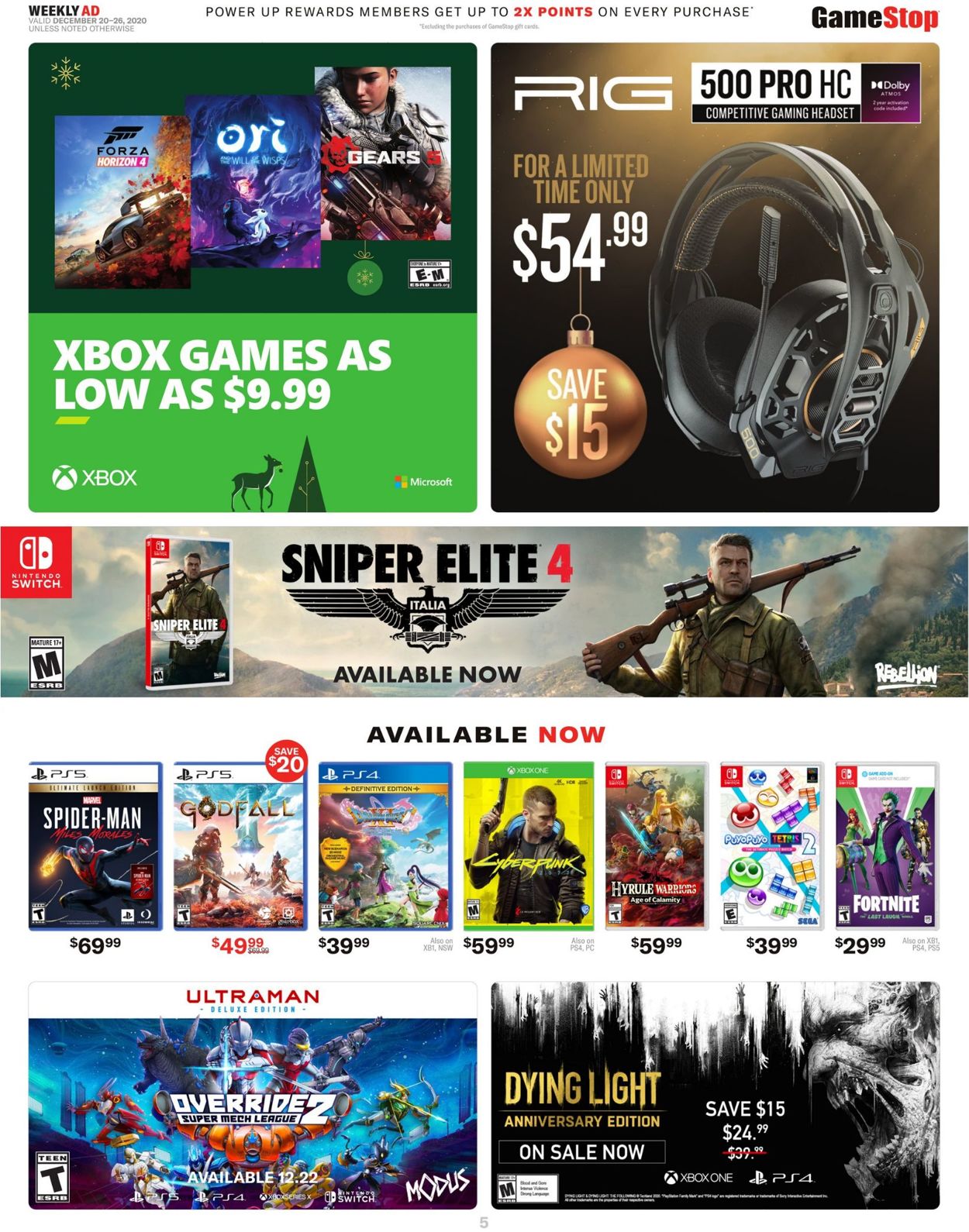The image showcases the weekly advertisement from GameStop, depicted on a white piece of paper. 

At the top left, the bold text "Weekly Ad" is prominently displayed. Centered at the top, a headline reads, "PowerUp Rewards members get up to 2X points on every purchase," emphasizing the benefits for members. On the top right, the iconic GameStop logo is visible.

Beneath the "Weekly Ad" headline, a green box on the top left side announces, "Xbox games as low as $9.99." Featured within this offer are titles such as Forza Horizon 4, Ori and the Will of the Wisps, and Gears 5. To the right of this section, there is an advertisement for a RIG gaming headset.

In the bottom center of the ad, an eye-catching promotion for "Sniper Elite 4," available on the Nintendo Switch, is displayed. Below this, various other games marked "available now" are listed. This lineup includes:
- Spider-Man: Miles Morales and Godfall for PS5
- Cyberpunk 2077 for Xbox One
- Hyrule Warriors and Fortnite for Nintendo Switch
- An additional, unidentified game for Nintendo Switch

Finally, at the very bottom of the ad, "Override 2" and "Dying Light: Anniversary Edition" are highlighted, rounding out the extensive offerings in this week's GameStop ad.